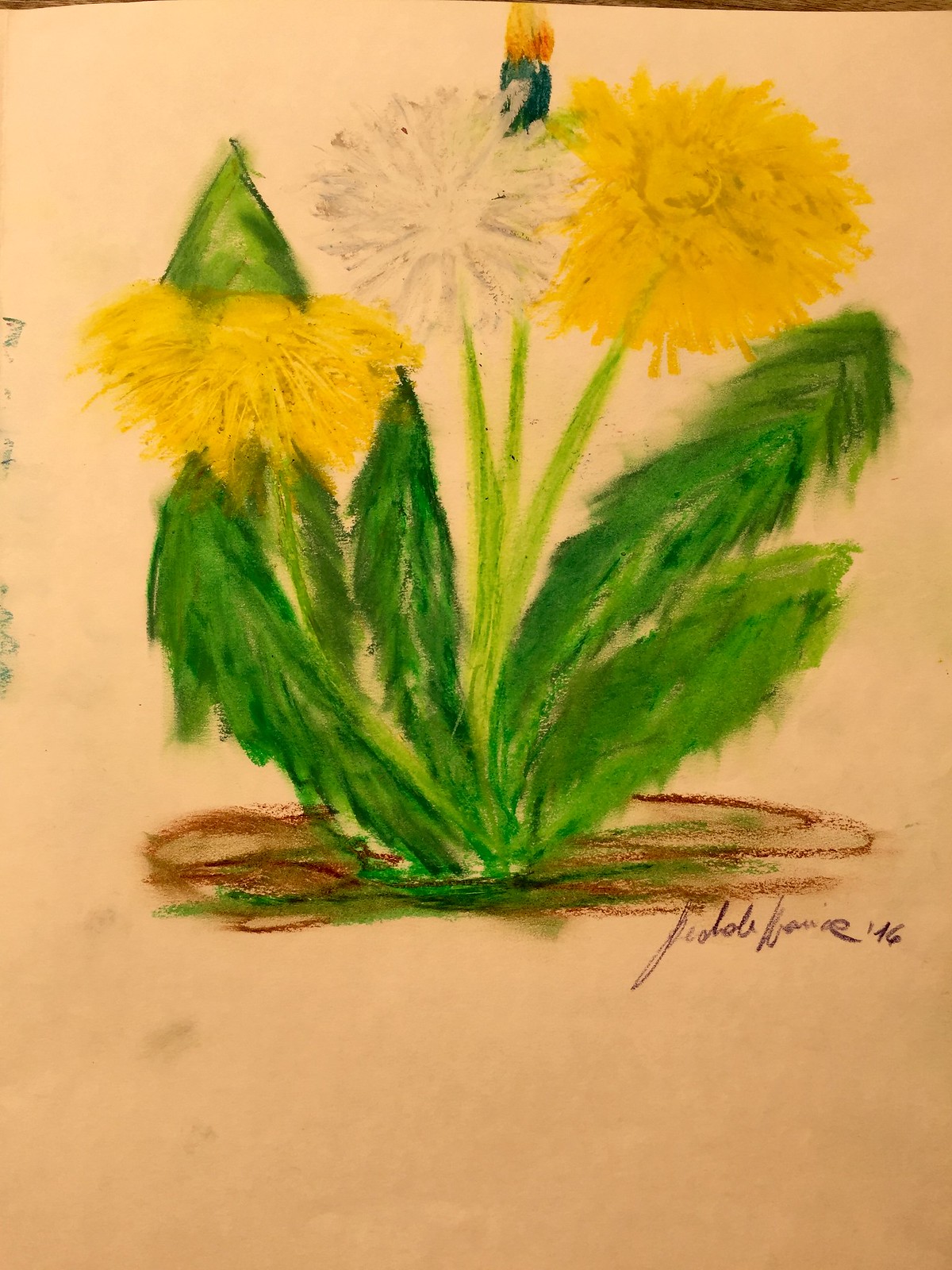This is a somewhat messy and blurry pastel drawing, potentially created with crayon or oil-based crayons, depicting a cluster of dandelions. There are three dandelions in various stages—two in yellow bloom and one that has gone to seed with white, fluffy seed pods, characteristically known for blowing to make a wish. The flowers are accompanied by six or seven green, smudgy leaves that have a furry texture and thin lime green stems, giving an almost pine tree-like appearance. There is a brown and green dirt area representing the ground at the base of the plant.

The majority of the illustration is concentrated in the top half of the page, set against a white background. However, the lighting causes it to appear slightly pink and yellowish. Additionally, the drawing features colorful smears towards the top, including a blot of blue, smears of yellow, and a small smudge of orange situated behind the gone-to-seed dandelion.

The piece also features two different signatures that pose some confusion about its origin: one, a childlike and sloppy signature dated “2016,” and the other, a more swoopy, adult-looking signature dated "'46", suggesting the year 1946. These elements contribute to the overall ambiguous nature of the artwork, making it appear both amateur and historical.